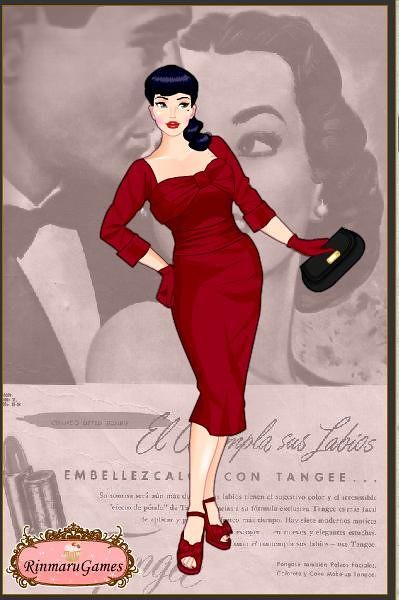The digital advertisement poster, evocative of a 1930s or 40s classic movie, features a striking composition of both black-and-white and vivid colors. In the background, a black-and-white image reminiscent of an old-time romantic film showcases a man in a tuxedo and bow tie, standing slightly behind a woman dressed in a fancy sleeveless gown, her hair elegantly styled into pin curls gathered into a bun at the back of her head, adorned with white pearl earrings. The woman gazes back at the man, adding to the nostalgic romantic aura.

Dominating the foreground is a brightly colored, cartoon figure of a dark-haired woman with heavy bangs, wearing a form-fitting red dress with three-quarter sleeves, matching red gloves, red platform shoes, and carrying a black clutch handbag. Her vivid red lipstick, matching the dress, highlights her beauty mark under her left eye. At the bottom left corner of the poster is an emblem reading "Minmaru Games" or "Remaru Games," alongside a tube of lipstick, underscoring the advertisement's focus on the red lipstick. The text in the background appears to be in Spanish, giving a noir romance feel, suggestive of a lipstick advertisement intertwined with classic cinema romance.